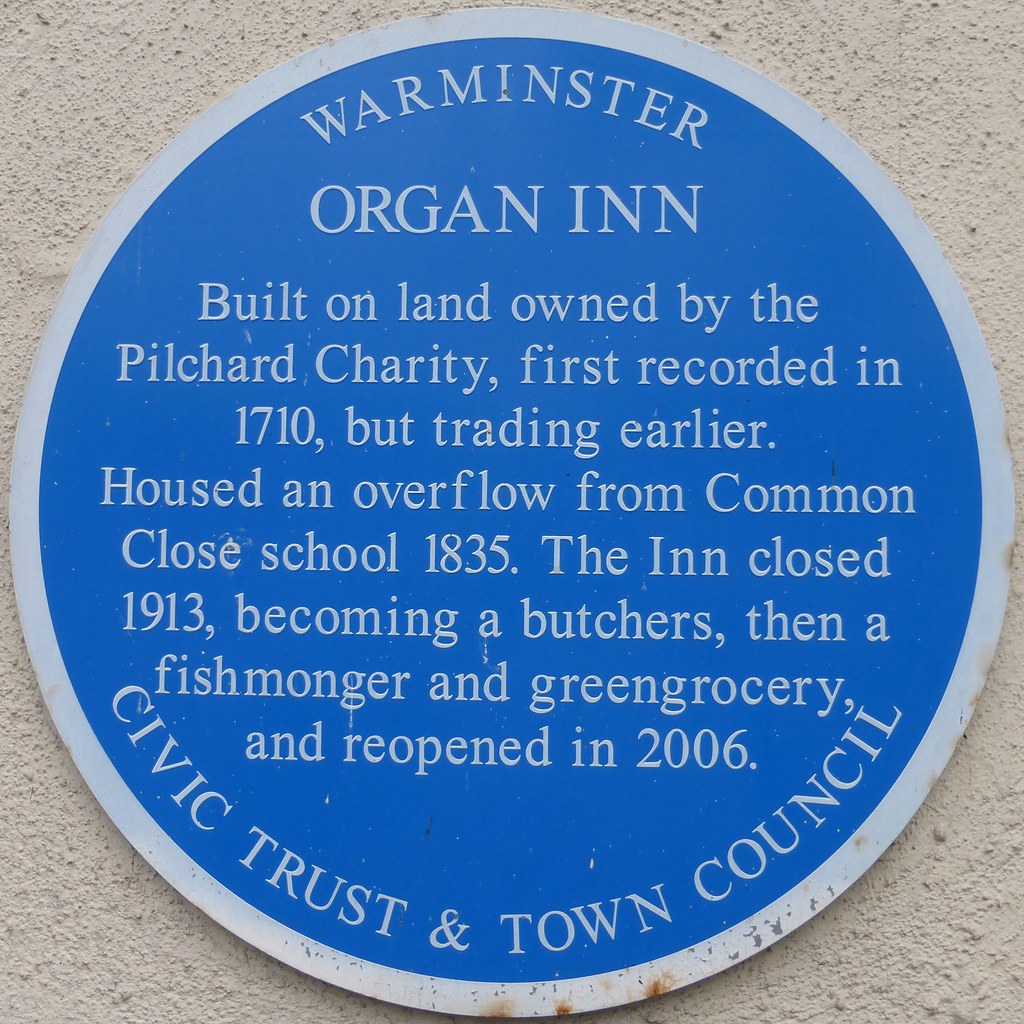The image depicts a round, gray metal sign attached to a somewhat dirty, white cement wall. The sign features a gray outline with a blue background inside. The text on the sign is white and straightforward. At the top of the circle, following its contour, is the word "Warminster," and at the bottom, also following the circle's edge, it reads "Civic Trust and Town Council." Centrally placed, in larger, all-capital letters, are the words "Organ Inn." Below this, in smaller text, the sign states: "Built on land owned by the Pilcher Charity, first recorded in 1710, but trading earlier. Housed an overflow from Common Close School in 1835. The inn closed in 1913, becoming a butcher's, then a fishmonger and green grocery, and reopened in 2006."